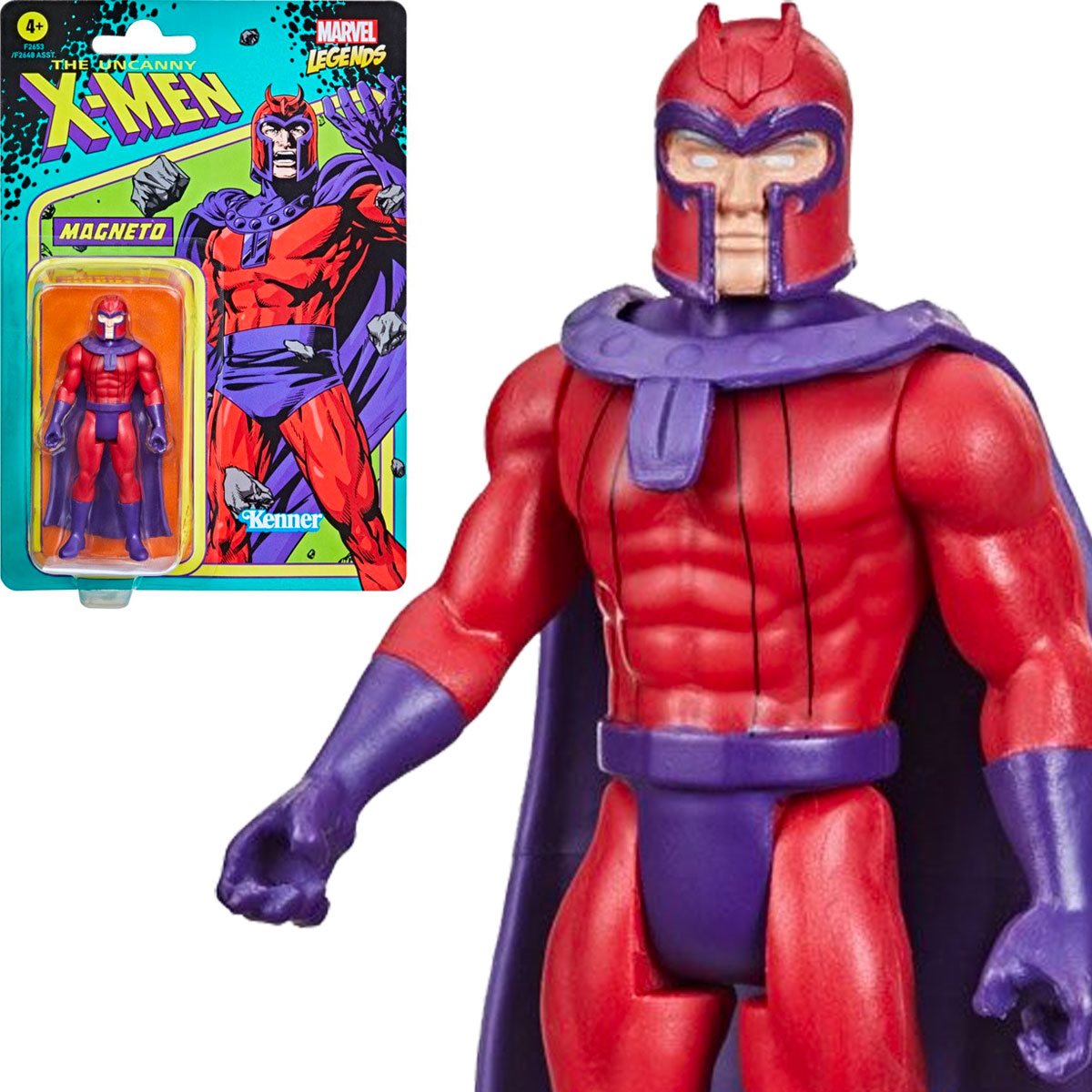This image depicts a detailed and vibrant action figure from the X-Men series, specifically of the character Magneto. On the left-hand side, the figure is shown inside its original packaging, which prominently features the titles "The Uncanny X-Men" in a yellowish-green font and "Marvel Legends" in the top right corner. The Kenner logo is displayed in blue and white lettering at the bottom of the box, which is primarily blue and green with rock graphics flying around. The action figure is enclosed in a clear plastic case, exhibiting Magneto's iconic outfit: a red body suit complemented by purple gloves, a centurion-style helmet with purple accents, a flowing purple cape, and a purple loincloth. Additional details emphasize his muscular build, including well-defined legs and a six-pack. To the right side of the packaging, there's a close-up art depiction of Magneto capturing the character's formidable and powerful stance. The figure is labeled suitable for ages four and up.